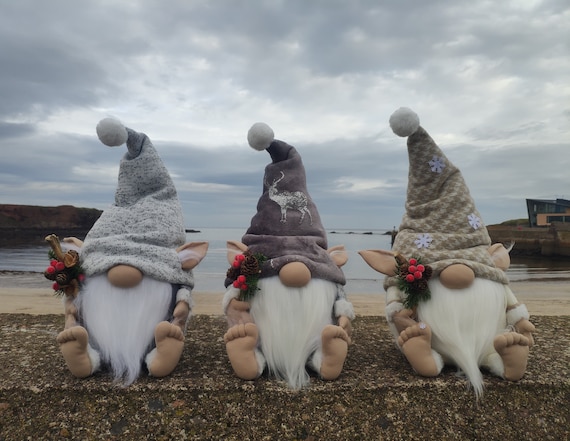In this photograph, three gnome statues sit side-by-side on a raised stone or concrete wall along the coastline. The gnomes, all with long, white, bushy beards and tall hats, obscure their eyes beneath the brims. Each features prominent elf-like ears and noses, with their bare feet visible. The gnome on the left wears a simple gray hat. The middle gnome sports a darker gray hat adorned with a white deer, as well as mistletoe on the right side of its face. The gnome on the right has a tan hat decorated with little snowflakes and also features mistletoe. The backdrop consists of a gloomy, cloud-filled sky over a beach, with a small house visible to the right.